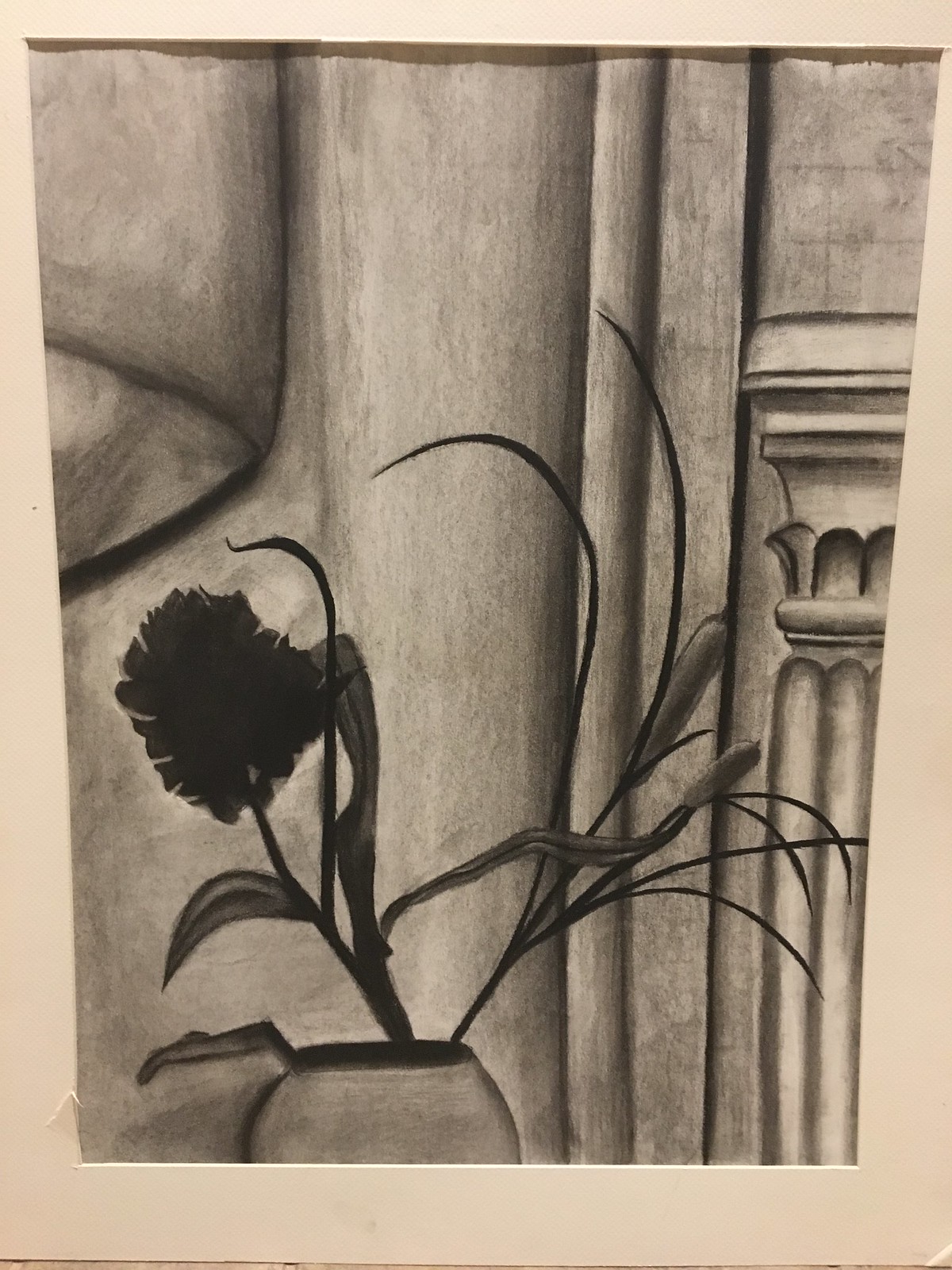This black-and-white drawing captures a detailed flower blooming from a partially visible vase, set against a creamy colored, matted background. The flower, rendered with numerous intricate petals, appears almost black in the monochromatic scheme. Its long, narrow stem and leaves add elegance to the composition. To the right, a meticulously drawn pillar stands, suggesting architectural elements, while a textured stone wall in the background adds depth and contrast to the scene.